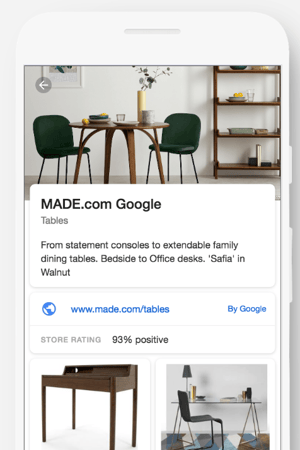The image is a screenshot of a Google search result. 

At the very top, there's a prominent image displaying a small dining table set for two, positioned within a cozy living room. Above this image, there is a black back arrow in the top left corner. To the side of the table, a bookshelf or rack holding additional plates and glassware is noticeable, contributing to the inviting ambiance of the space.

Below the main image, large text reads "MADE.COM," with "MADE" written in all capital letters. Underneath, a subtitle in smaller gray text mentions "Assist tables in dark gray." 

Following this, a black text description details various types of tables available: "From statement consoles to extendable family dining tables, bedside to office desks. Office desks in Safiyan walnut."

The link "www.made.com/tables" is displayed in blue text alongside another blue text link labeled "Google." An accompanying image of a globe is situated beside the link.

Beneath this, the store rating is shown as "93% positive."

Below this description, there are two additional images of tables; one depicts a wooden brown table, while the other features a glass table with a modern plastic chair placed on a geometric patterned mat. The clear table hosts a small lamp and a few cups and plates, although these details are somewhat blurry.

Overall, the Google search result presents an inviting array of dining and office table options with a direct link to the MADE.COM website.